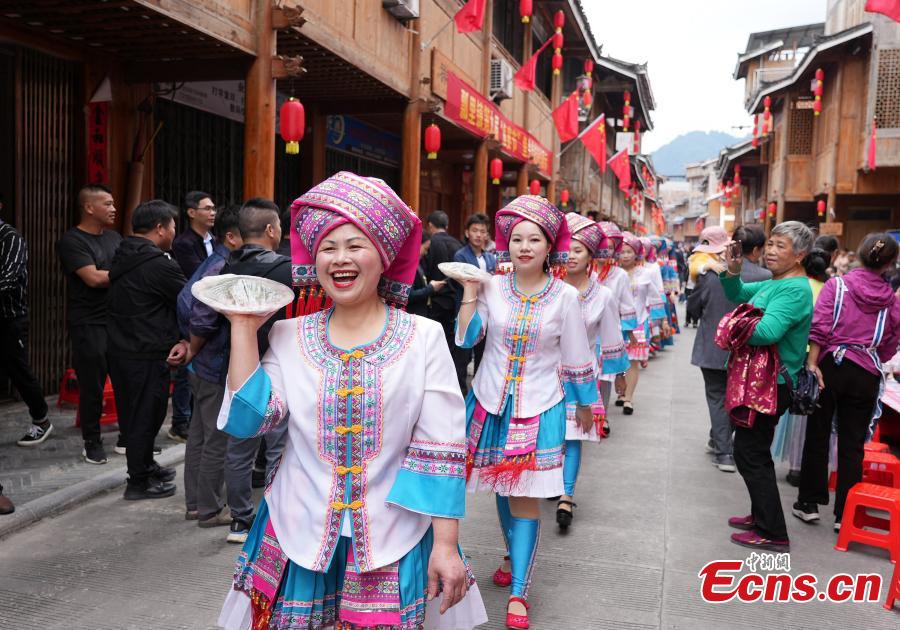The image captures a vibrant outdoor parade, possibly during a carnival or festival, set in an Asian locale, suggested by the traditional Chinese and Asian influences present throughout the scene. In the foreground, a line of women marches in unison, each dressed in white traditional garb accented with pink and blue trimmings. They wear matching pink turbans styled like headgear, imbuing the scene with a striking uniformity. The women appear joyous, laughing as they hold silver balls, or plates, up in their right hands, reminiscent of waitresses carrying trays. The street is lined with onlookers, standing on both sides, closely observing the parade. The surroundings are bustling, indicative of a busy shopping street with buildings decked in red flags and Chinese lanterns, enhancing the festive atmosphere. A banner with Chinese characters hangs prominently, while in the bottom right corner of the photograph, the text "ECNS.CN" is visible.